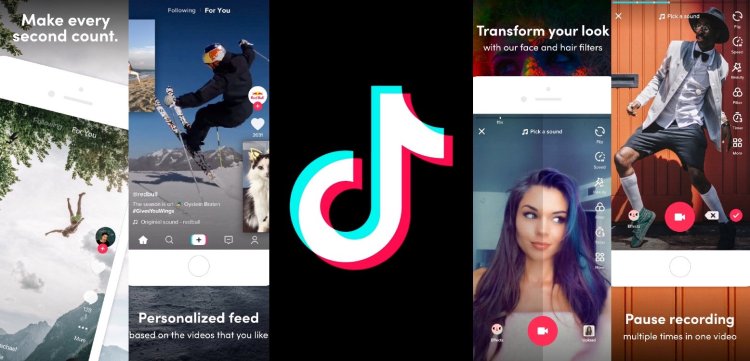The image depicts a detailed layout of a TikTok page, divided into five distinct sections:

1. **Left Section:** The phrase "Make every second count" overlays an image of a skydiver, emphasizing the importance of seizing every moment.

2. **Second Section:** A skier dressed in a black ski outfit navigates snowy mountains in the background. At the very bottom, the text "Personalized feed based on the videos that you like" appears on a gray background.

3. **Central Section:** Occupying the middle of the layout is the TikTok logo displayed prominently against a black background, featuring its signature green, blue, white, and red colors.

4. **Fourth Section:** Under the header "Transform your look," a girl showcases various hair colors—black, purple, and blue—demonstrating the platform's face and hair filters. Below her image, there is a camera icon within a red circle, ready for activation.

5. **Rightmost Section:** A stylishly dressed man stands, wearing gray shorts, white socks, gray tennis shoes, a white shirt with a black bow tie, a light gray blazer, glasses, and a black fedora hat. His right side is lined with six clickable icons, offering diverse functionalities. At the bottom, there's a red circle with a white camera inside it, adjacent to a plain white bar with a gray circle in it, and the text "Pause recording multiple times in one video" prominently displayed.

This comprehensive layout illustrates TikTok's user interface, highlighting its interactive features and diverse content creation tools.